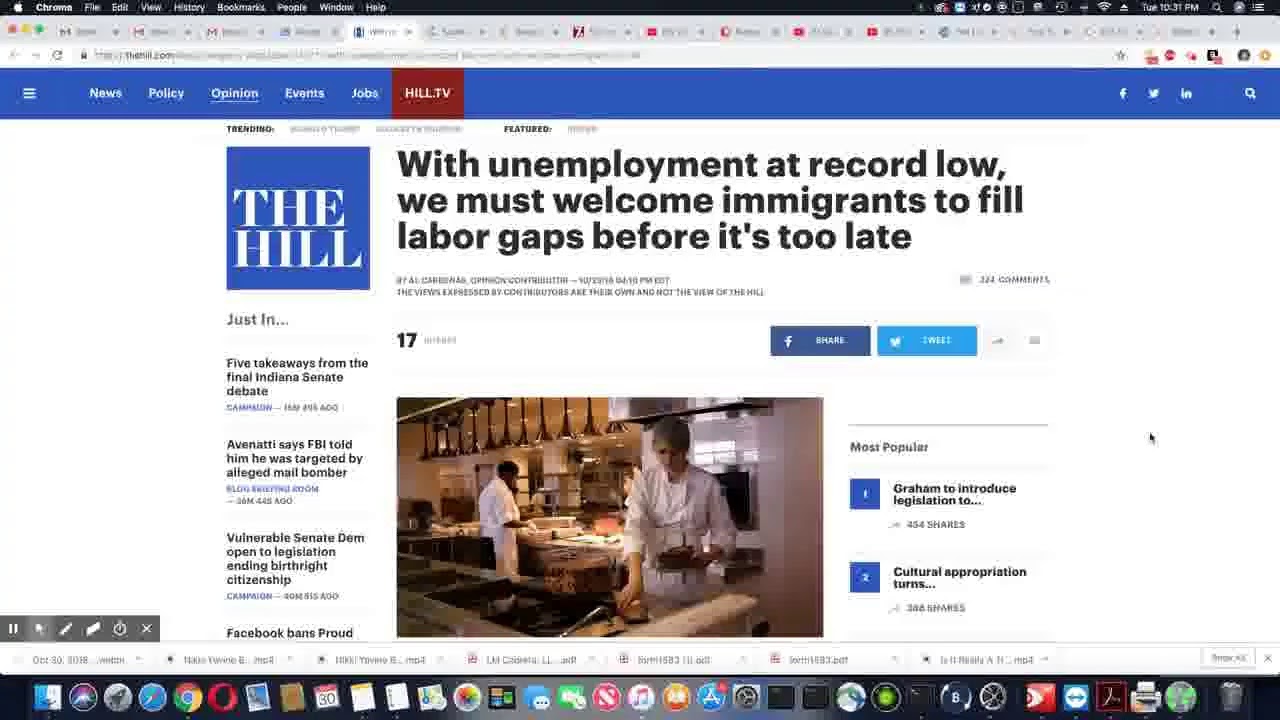The screenshot displays a website viewed via the Chrome browser, as indicated by the browser's interface at the top. The top menu bar includes standard options such as File, Edit, View, History, Bookmarks, People, Window, and Help. The image quality is rather poor, making it challenging to discern details clearly across the interface. The address bar is also blurry, obscuring the precise URL. The browser appears to have multiple tabs open, though their contents are not identifiable.

The website shown is The Hill, a news outlet. At the top of the site is a blue navigation bar containing several menu options: a burger menu icon on the left, followed by tabs labeled News, Policy, Opinion, Events, Jobs, and Hill TV. The Hill's logo, a square blue box with white text, is situated in the top left corner. The main article displayed is headline: "With unemployment at record low, we must welcome immigrants to fill labor gaps before it's too late." Below the article's headline, there's a photograph depicting people working in a kitchen, presumably related to the article's content.